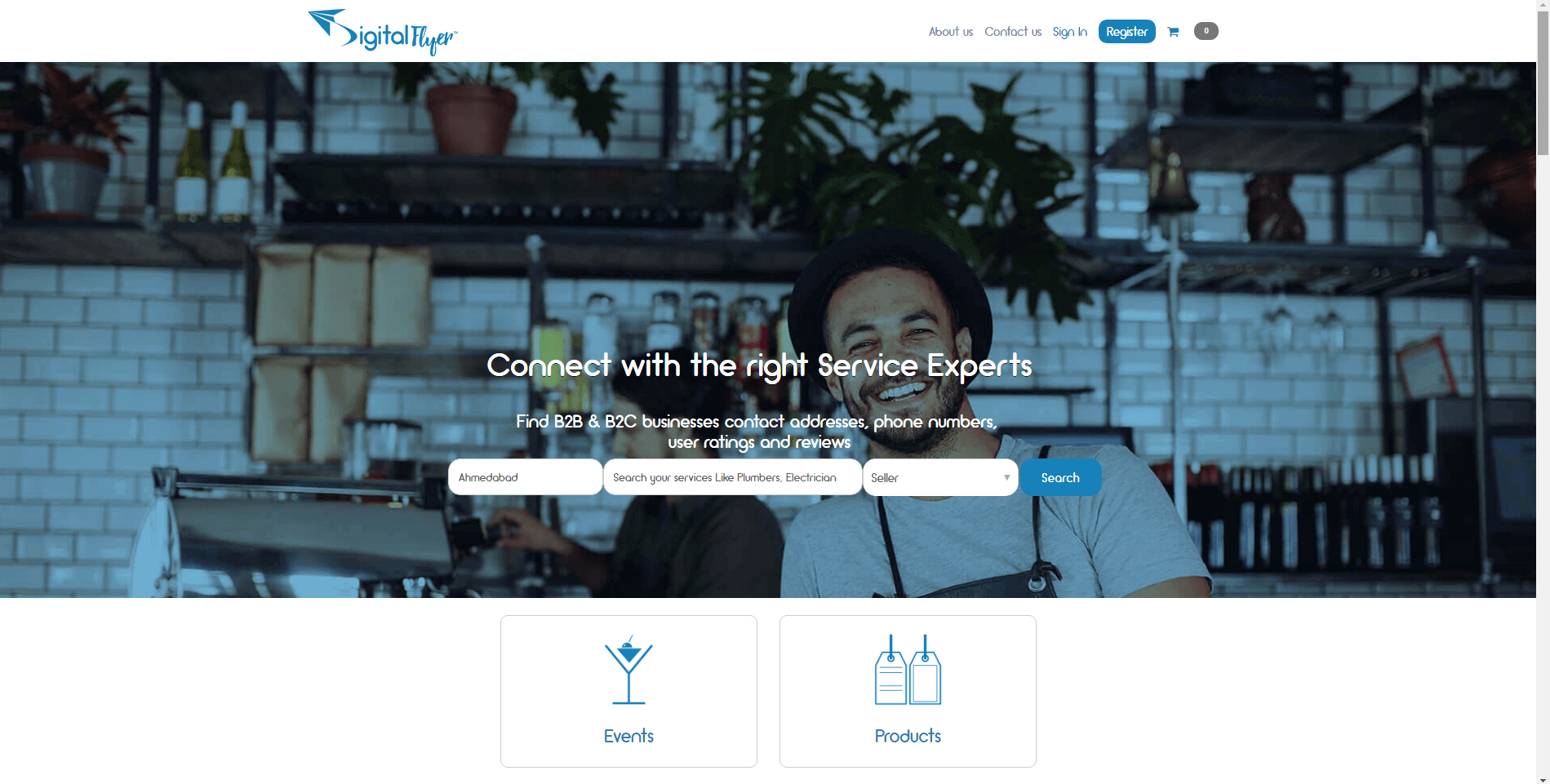The image depicts a website dedicated to digital flyers. The site name, "DIGITAL FLYER," is prominently displayed with a stylized logo that incorporates an airplane graphic followed by a graceful swoosh. On the right-hand side of the webpage, navigation links for "About Us," "Contact Us," and "Sign In" are clearly visible, alongside an oval-shaped "Register" button. Additionally, there are icons for a shopping cart and a user profile, set against the backdrop of a scroll bar located at the very top of the page.

The main image featured on the website is of a cheerful man wearing a hat with a rounded brim, seemingly seated in a cozy bistro. The background includes a white brick wall with text that reads, "Connect with the Right Service Experts." Below this headline, there is a brief description offering details about finding B2B and B2C business contacts, addresses, phone numbers, user ratings, and reviews, though some of the smaller text is difficult to decipher.

Further down the page, there are three oval-shaped boxes; the central one is noticeably longer than the others, but the text within them is not clearly readable. Next to these boxes, there is a blue search bar. The section below highlights "Events" and "Products," each represented by two respective icons.